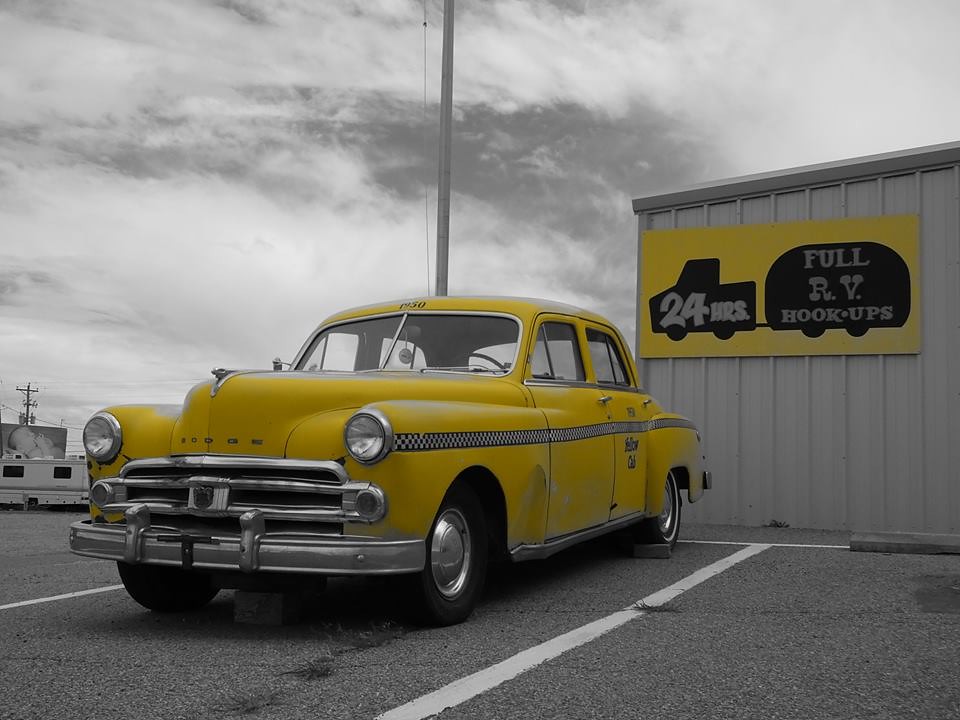The image depicts an old yellow Dodge taxi from the 60s or 70s era, parked outdoors during the daytime. The rectangular photograph, wider than it is tall, captures the front and right side of the cab, which features chrome fenders and a grill, along with round headlights. Notably, it lacks the typical taxi sign on its roof. A distinctive black and white checkerboard pattern runs along the side of the vehicle, stretching from the front circular headlight to the rear taillight. On the rear door, the words "Yellow Cab" are displayed beneath the checkerboard stripe in black text. 

The taxi is parked on a gray paved area marked with white lines. To the right, there's a gray metal building with a yellow sign that has a black outline of a truck pulling an RV. The sign reads "24 hours" in silver on the truck, and "Full RV hookups" on the RV. The sky above is large and gray, filled with giant white clouds. The entire image is in black and white, except for the vibrant yellow taxi and the yellow sign, adding a striking contrast to the scene.